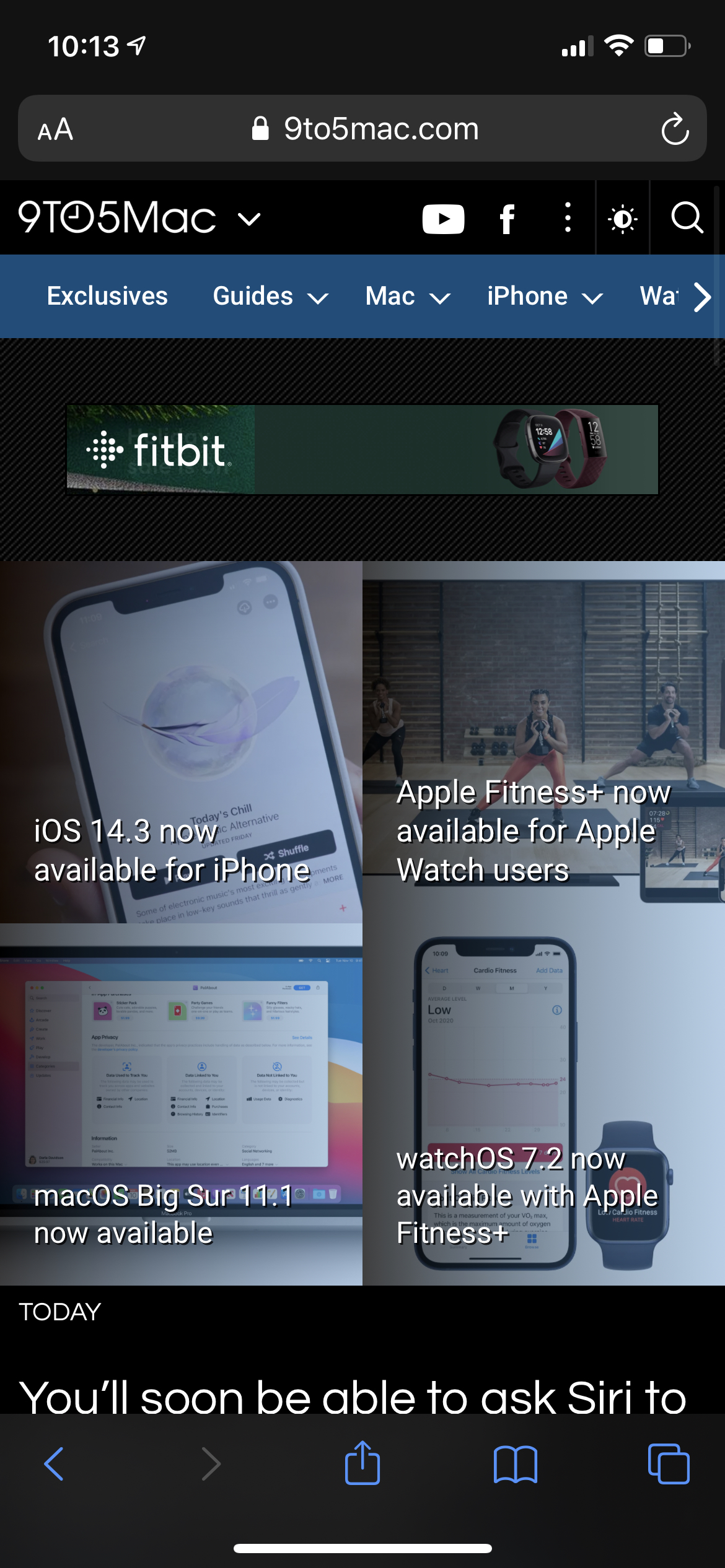The image is a screenshot of an iPhone displaying a webpage from the website 9to5mac.com. The time on the phone is 10:13, and the device has around 50% battery remaining with a full Wi-Fi signal. The user is browsing the webpage to find information on various versions of macOS. 

There is a prominent notification alert indicating that iOS 14.3 is available for download on the device. Additionally, the screenshot reveals information about macOS Big Sur 11.1, along with updates for the Apple Watch and Apple Fitness. The webpage is well-organized, providing a comprehensive overview of upcoming software updates across multiple Apple products.